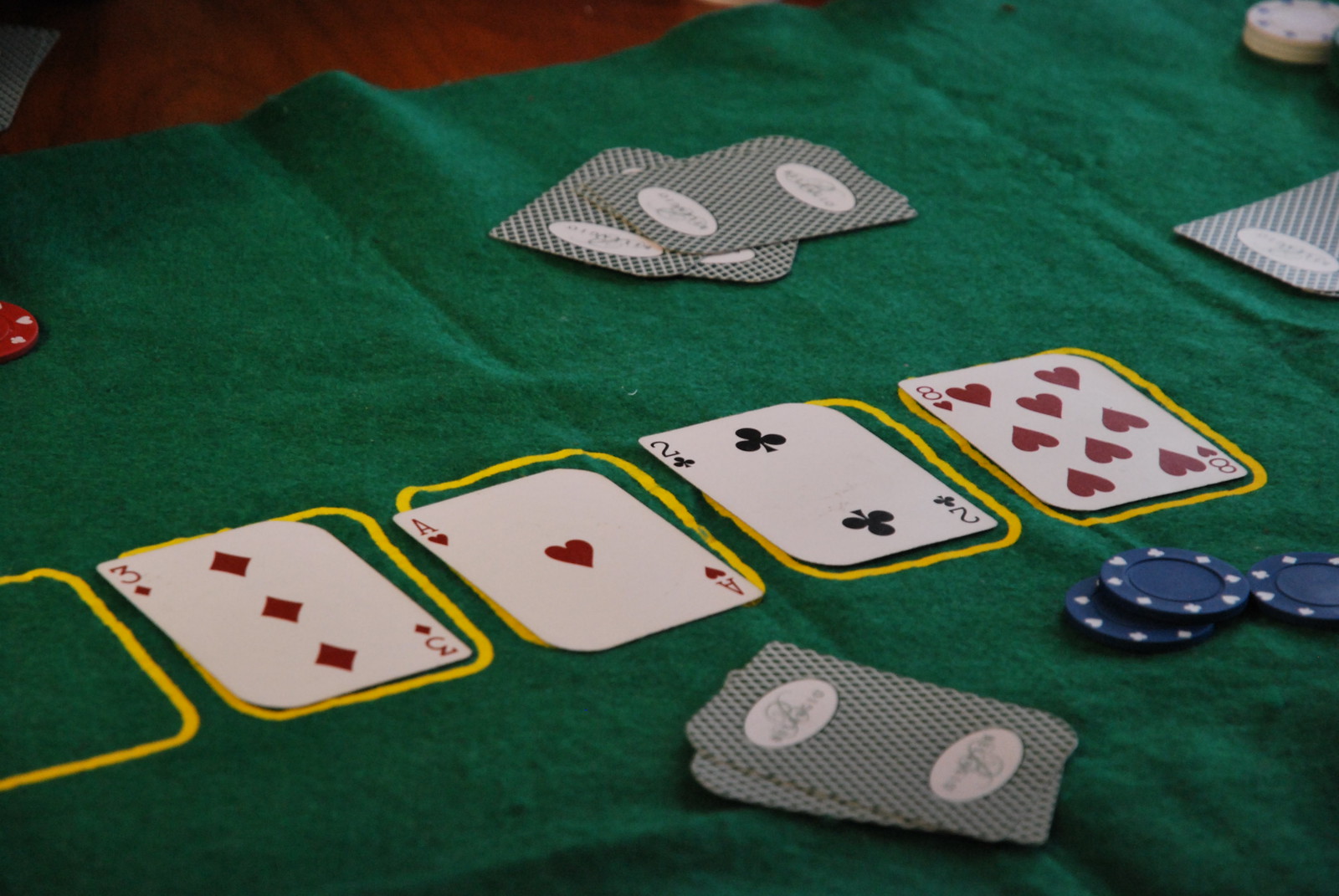The image is an indoor, close-up photograph of a game mat specifically designed for playing cards. The green mat lies on a wooden table, part of which is visible in the upper left corner of the image. Diagonally placed from the left towards the center-right, the mat features yellow card outlines, with four playing cards placed within them. The cards, aligned left to right, are the three of diamonds, ace of hearts, two of clubs, and another ace of hearts. Below these cards, there is a small deck with a distinctive black checkered pattern and white ovals on the sides. To the right and slightly above this deck, three poker chips, either green or blue with white spots along their edges, are positioned—two chips are stacked, and one lies separately to their right.

In the upper center of the background, five or six more playing cards, all face down with the same back design, are scattered; some are vertical while others are slightly diagonal. In the upper right corner and just below it, a part of a playing card intrudes into the frame. Similarly, along the left edge, a segment of a red poker chip is visible. The photograph contains no text or printed words.